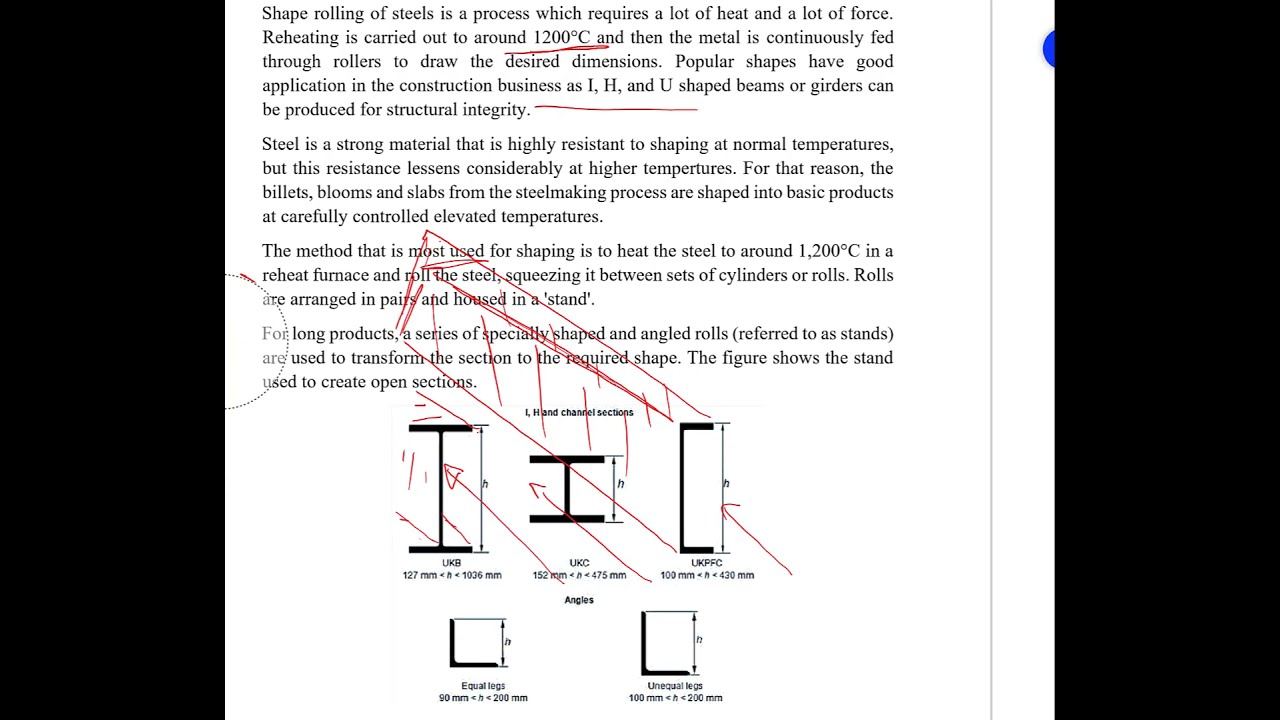This horizontally rectangular image features a page from a textbook or webpage, bordered by solid black margins on either side. The central content consists of four left-aligned paragraphs discussing the process of shape rolling of steels, which requires significant heat and force, specifically mentioning 1200 degrees Celsius. Several annotations in red ink are visible, with important terms like "1200 degrees Celsius" and "business as I, H, and U" underlined. Towards the bottom, a detailed, computer-generated diagram illustrates various steel angles and dimensions (90 mm, 100 mm, 152 mm). This diagram is further annotated with red hand-drawn lines and arrows, indicating measurements and different perspectives of steel components.